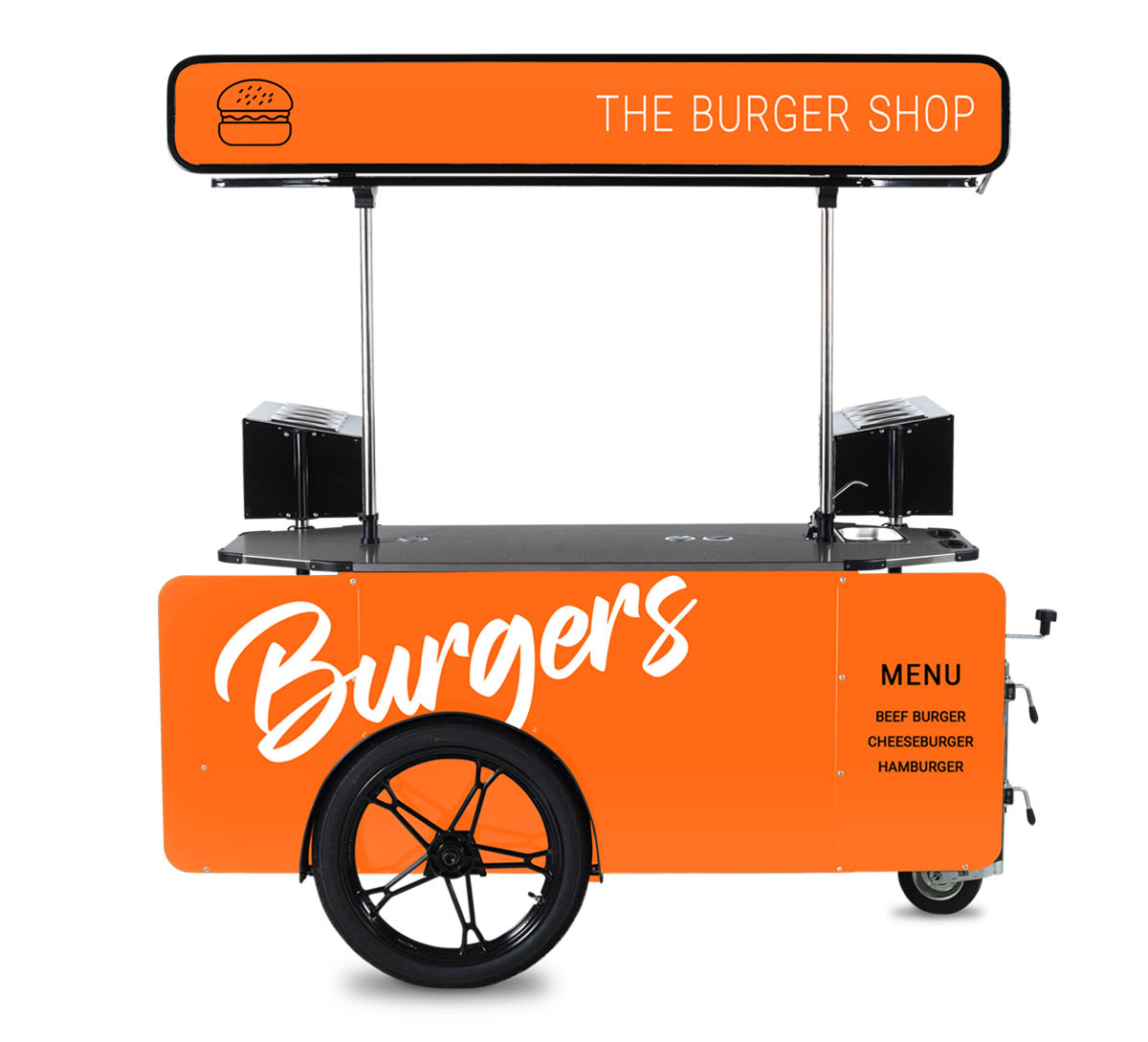The image features a minimal, lightweight, portable burger cart designed to be towed by a bicycle, resembling a hot dog stand. The cart is primarily orange, with white and black accents. Prominently displayed in white letters on its orange facade is the name "The Burger Shop," complemented by a graphic of a burger. Below this, the main sign states "burgers" in large white font, while off to the side, a black sign with white writing reads "menu," listing options such as beef burger, cheeseburger, and hamburger. The cart includes a black countertop, which might be equipped with cash registers or small ovens, and rests on two black tires. Handles on the right side imply functionality for towing or accessing storage compartments, though their exact purpose is unclear. The overall presentation suggests a product photo, showcasing the cart's design and potential customizability for different food stands.